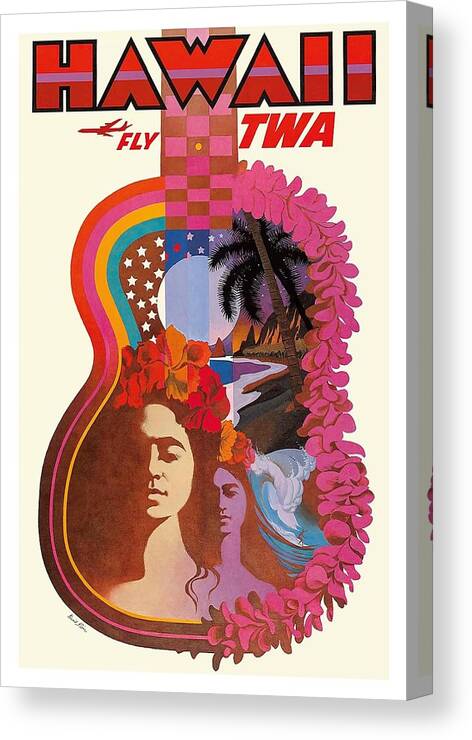The image appears to be a vibrant and detailed advertisement for TWA, promoting travel to Hawaii. At the top in bold letters, it reads "HAWAII," with a black outer border and a red interior, accentuated by a small purple stripe across the word. Below it, the phrase "FLY" in all caps is displayed alongside an airplane illustration, with "TWA" written in red italics to the right.

The centerpiece of the image is a meticulously painted ukulele, with the neck displaying a pink and brown checkerboard pattern. Surrounding the ukulele's body are colorful borders: yellow, blue, pink, and red lines on the left side, and flowers forming a lei on the right, which add to the Hawaiian theme.

On the body of the ukulele, there are intricate designs including a beach scene with waves, a palm tree, and two women adorned with flower crowns, suggesting a native Hawaiian setting. Additionally, the central hole of the ukulele is artistically depicted as the moon. Also visible is a surfboarder riding the waves, which furthers the allure of the tropical destination. The overall aesthetic is both inviting and exotic, capturing the captivating essence of Hawaii.